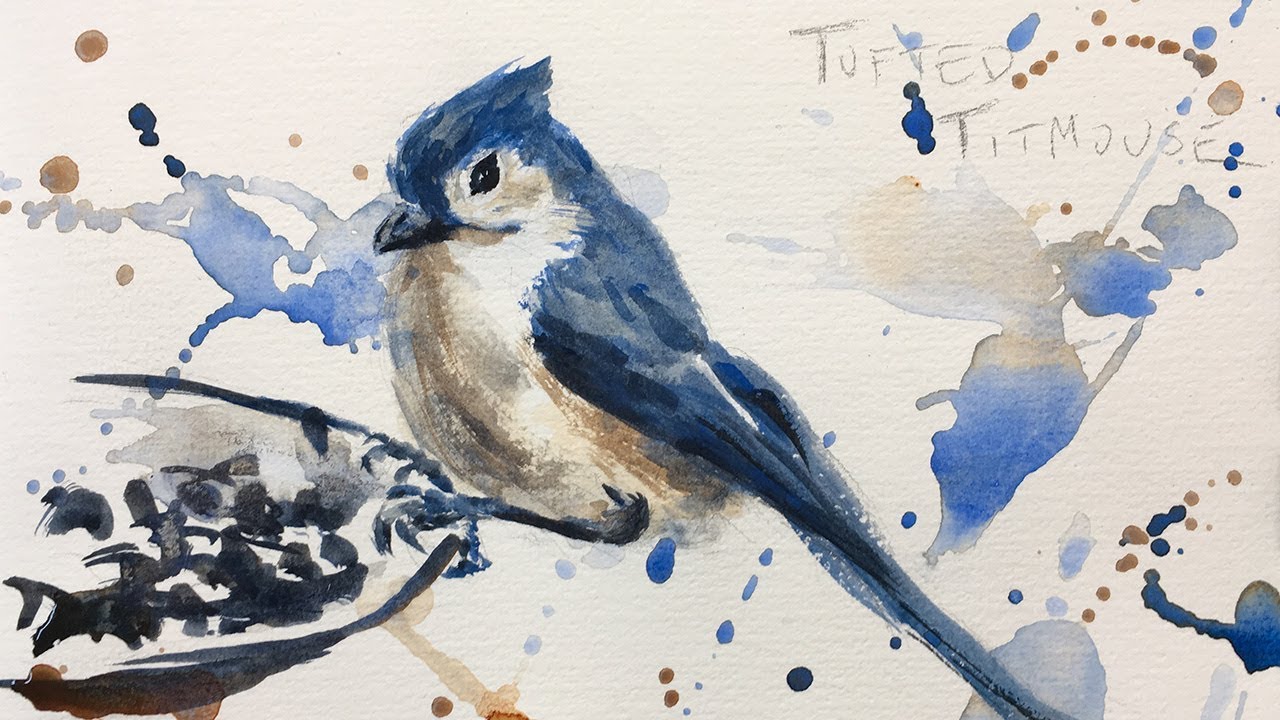This detailed watercolor painting portrays a bird, specifically identified as a Tufted Titmouse, based on the pencil inscription "Tufted Titmouse" located in the top right corner. The bird, which somewhat resembles a blue jay, is perched on the edge of a round, black bowl. The avian subject features a dark blue, almost grayish-blue, plumage that covers its body, transitioning into darker blue wings. It has black eyes and a small, black beak. The chest and belly of the bird are primarily white with hints of beige and gray for shading. The bird also boasts a long blue tail and blue feet. Surrounding the bird are loose, abstract splashes of watercolor paint in shades of blue and brown, which blend seamlessly into the white paper background, adding an ethereal, free-flowing quality to the artwork.